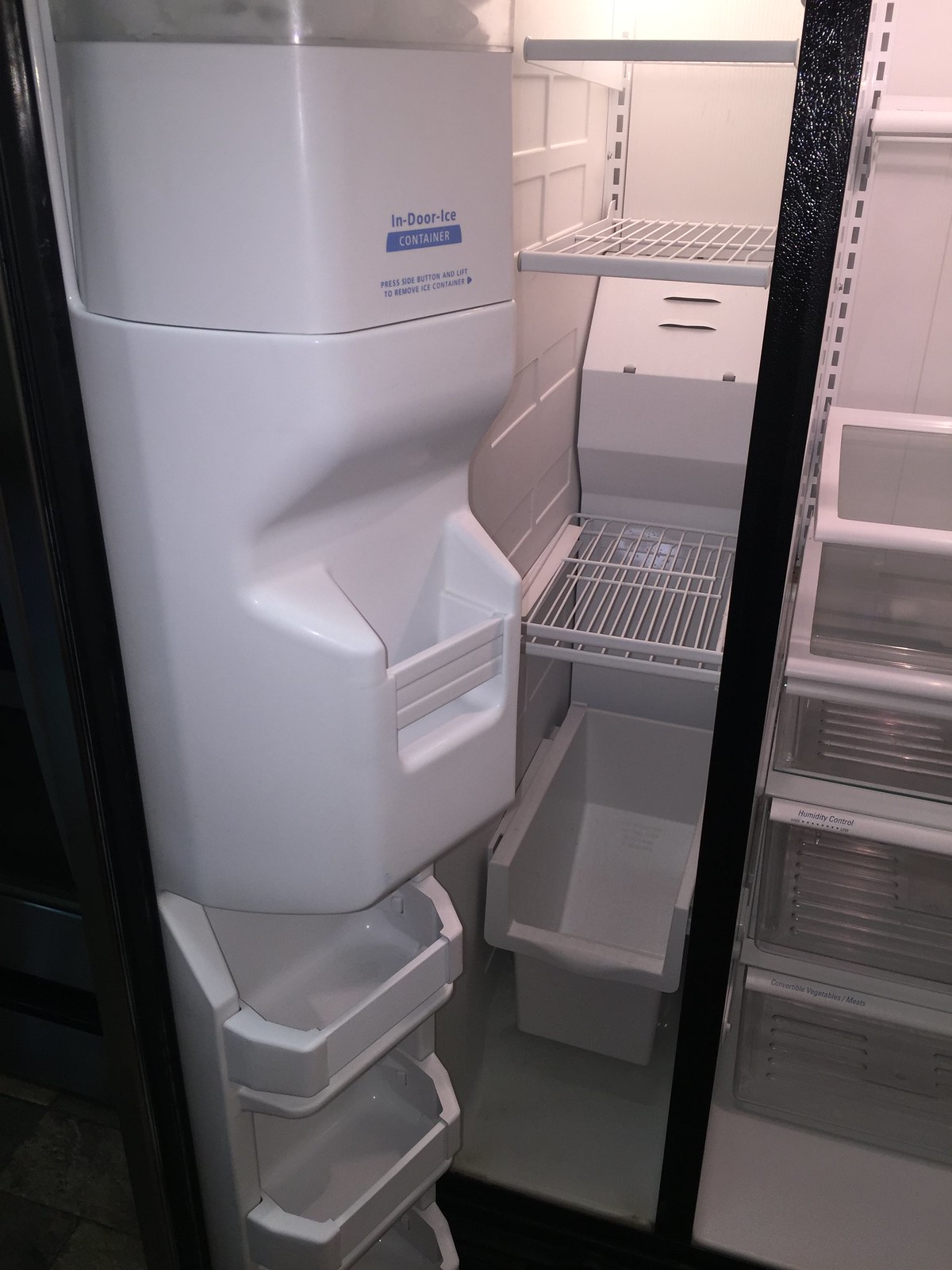This detailed color photograph captures the open interior of a side-by-side refrigerator and freezer. The left side, which is the freezer, is predominantly featured with its vertical layout. The freezer door exhibits multiple molded white plastic shelves and a transparent section at the top, where you can identify the indoor ice maker, clearly labeled with instructions for removal ("Press side button and lift to remove ice container"). The main compartment of the freezer includes adjustable white metal shelves set against a white backdrop, bathed in a yellow glow from the internal light. At the bottom, a white plastic bin serves as a storage container for frozen items. The right side of the image hints at the refrigerator section, which shows parts of glass shelving and a slight view of the door interiors, divided from the freezer by a thin vertical black strip.